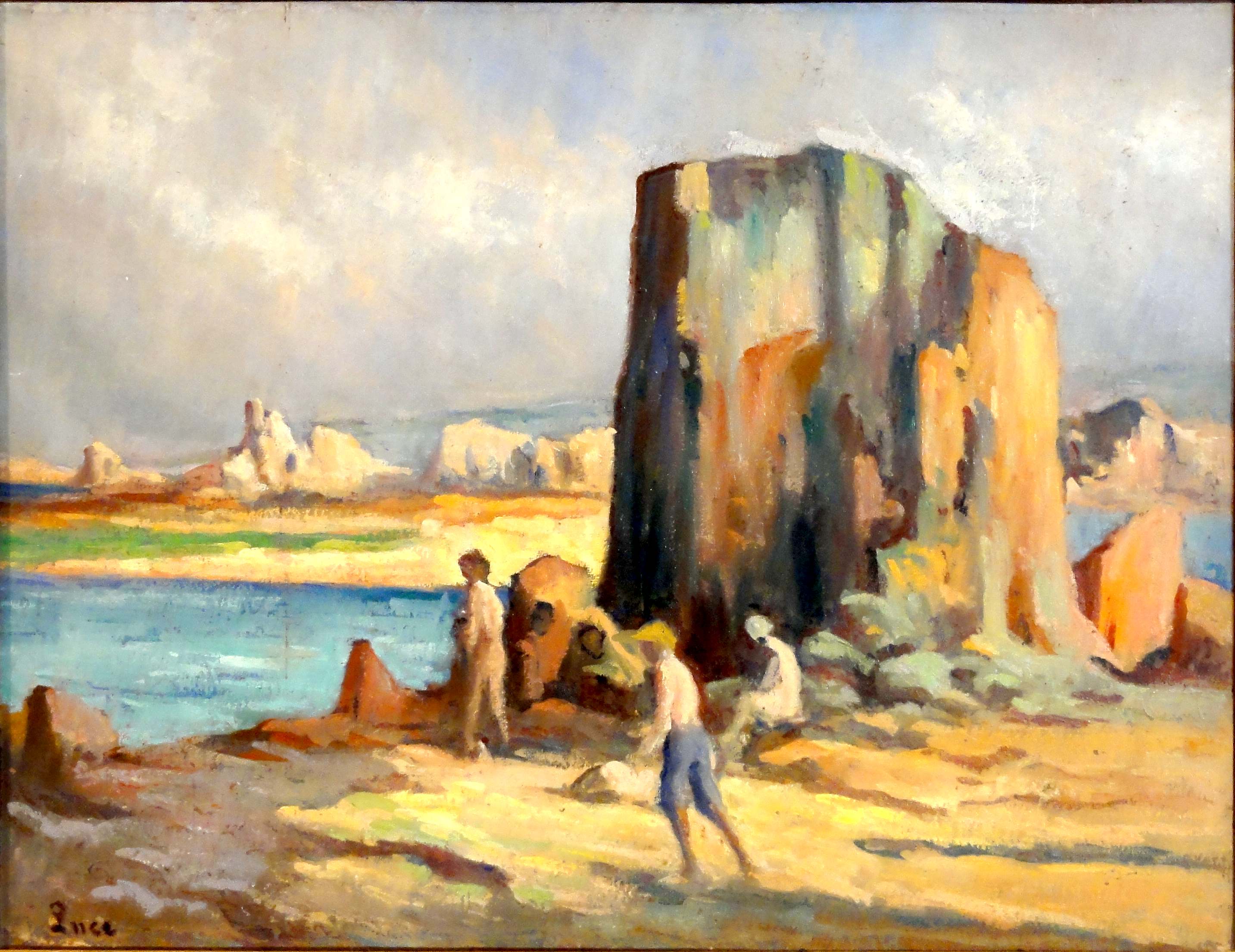This acrylic painting vividly captures an outdoor scene near a body of water, likely a lake, characterized by a mix of impressionistic and soft strokes lending it a slightly blurry effect. The focus is on three individuals standing at the water's edge. Notably, there are two boys, one older with brown hair, shirtless, and dressed in brown pants, and the other younger with blonde hair, shirtless, and wearing blue knee-length shorts. 

The left side of the painting features the deep blue waters of the lake, bordered by a shore that bursts with colors—white, pink, yellow, and orange—adding varied textures and vibrancy. A distinct standing rock formation is present in the immediate background, along with more scattered rock formations that appear as smaller mesas or flat-topped rocks rising from the ground. Further in the distance, a towering mountain range stretches above these rock formations.

The sky is predominantly overcast, presenting hues of gray and white clouds with only occasional patches of blue, contributing to a hazy atmosphere. A touch of green is discernible in the top left corner, and the lower left corner features the artist's signature, although it remains illegible. This painting captures the serene yet dynamic interplay between the natural elements—water, rock, and sky—against the human presence in this tranquil setting.